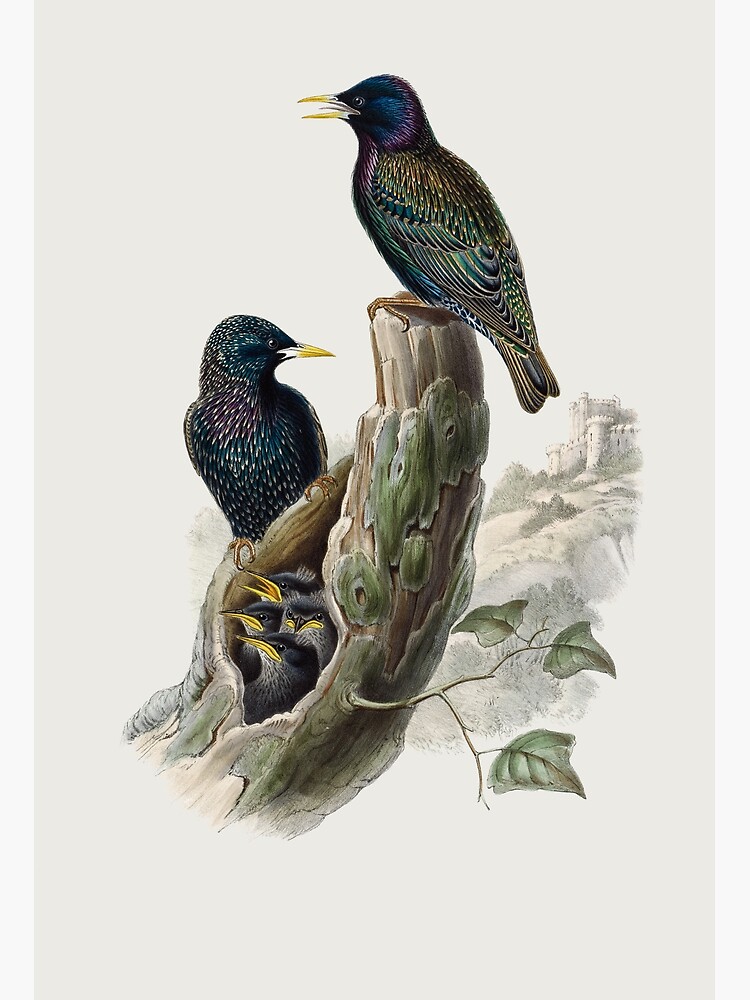This detailed and realistic drawing showcases a pair of iridescent black birds perched on an old tree limb, which holds their nest in a crevice. The parent birds, with their striking long yellow bills, display vibrant feathers that shimmer with hues of green, yellow, red, orange, purple, and blue against their predominantly black plumage. Nestled together, they attentively guard their four chicks, one of which has its mouth slightly open. The limb, while aged and weathered, still supports some leaves, suggesting resilience despite its abuse. The background features a white castle and a green hill, with the scene framed by thin white borders on either side. The composition artfully highlights the birds as the focal point, with the castle providing a picturesque backdrop.